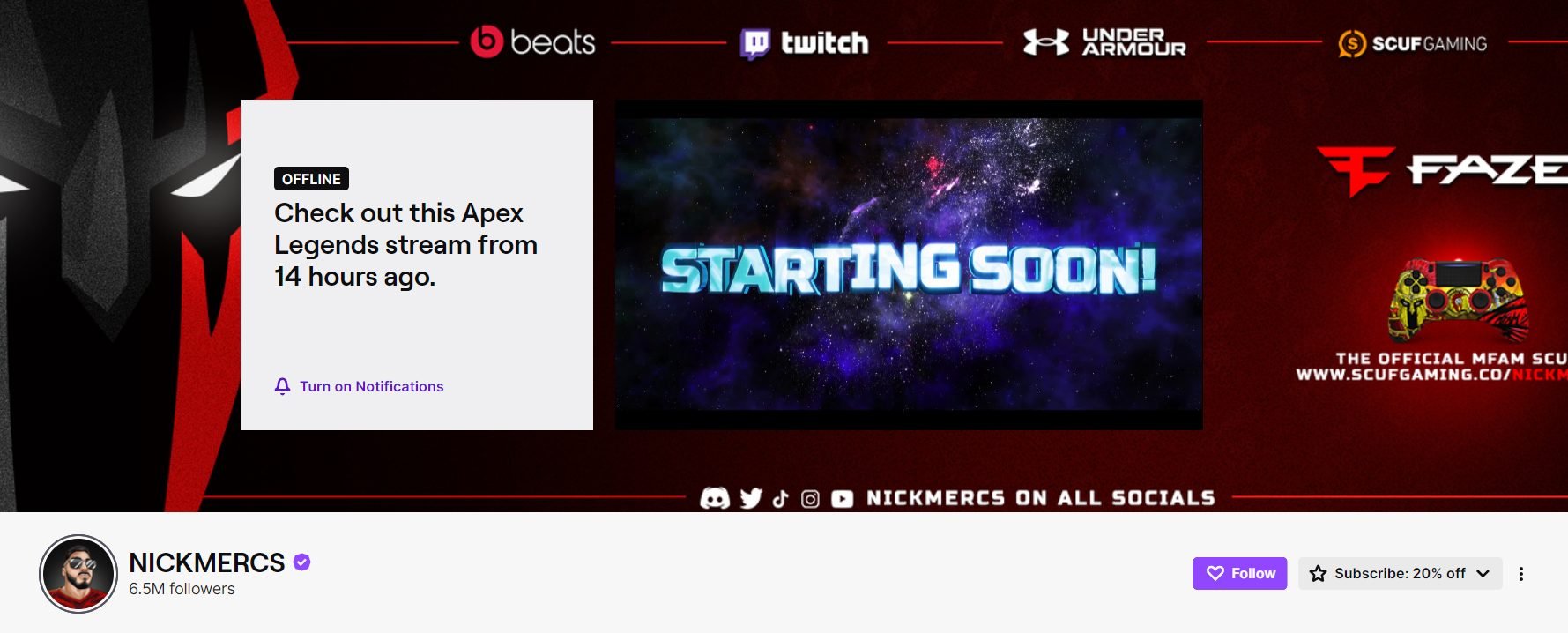This image depicts a web or landing page for a video game streaming channel. The main features of the page are richly detailed:

**Top Section:**
- The top of the page includes prominent brand icons for Beats, Twitch, Under Armour, and Scuf Gaming, indicating sponsorship or partnerships.

**Main Image:**
- Dominating the horizontal layout is a bold red background. On the far left, there is an image of a video game character with an intense expression. This close-up shot features a face with glowing eyes and a striking red and black mask, creating a sense of energy and suspense.

**Pop-Up Notification:**
- A white pop-up box towards the center of the layout announces that the stream is currently offline. It invites viewers to check out an APEX Legends stream from 14 hours ago.

**Middle Section:**
- The core of the page presents a video screen with text reading "Starting Soon." This text is set against a space-themed background, which adds a futuristic and exciting feel to the streaming experience.

**Right Section:**
- Positioned to the right of the video screen is the Faze logo, a well-known esports organization. Below the logo, there is an image of a vibrant red and yellow game controller, possibly indicating the streamer’s preferred gaming equipment.

**Footer Information:**
- At the bottom, there is a text that states "Nick Merck's 6.5 million followers," highlighting the popularity and substantial following of the streamer. This indicates that the page likely belongs to Nick Merck, a prominent figure in the streaming community.

The combination of brand logos, character imagery, futuristic themes, and follower count suggests a high-profile, professional gaming channel designed to attract and engage a substantial audience.